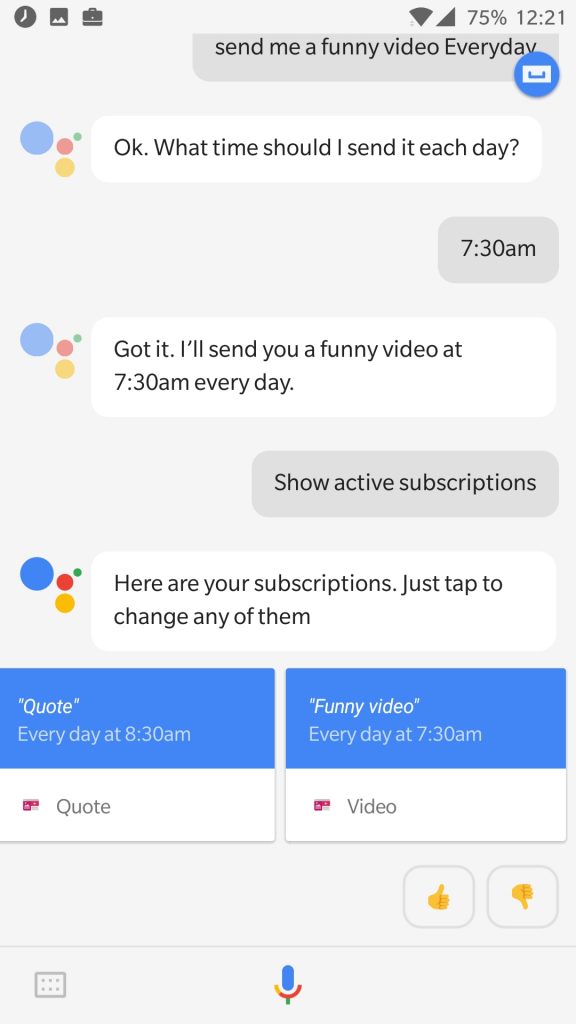The image depicts a cell phone screen showcasing a chat conversation with an AI. On the upper-left corner, a clock icon is followed by a picture icon, a suitcase icon, and several indicators on the right: Wi-Fi signal, cellular bars, a 75% battery charge, and the time 12:21.

The chat reveals a user requesting, "send me a funny video every day," to which the AI, represented by the Google AI logo (a colorful arrangement of blue, red, yellow, and green circles), responds, "Okay, what time should I send it each day?" The user specifies, "7:30 a.m.," and the AI confirms, "Got it, I'll send you a funny video at 7:30 a.m. every day."

Further into the conversation, the user asks the AI to "show active subscriptions." The AI replies, "Here are your subscriptions, just tap to change any of them." Below this, two rectangular subscription summaries are displayed. The first rectangle is labeled "quote," indicating a daily quote at 9:30 a.m., and the second rectangle is labeled "video," indicating a funny video at 7:30 a.m. Both rectangles have a blue upper section and a white lower section.

At the bottom right of the screen, there are yellow thumbs-up and thumbs-down icons for feedback, with a gray line beneath them. On the bottom left, two lines comprising three dots, enclosed in a gray outline, precede the Google Voice icon – a blue, yellow, red, and green microphone – located in the middle.